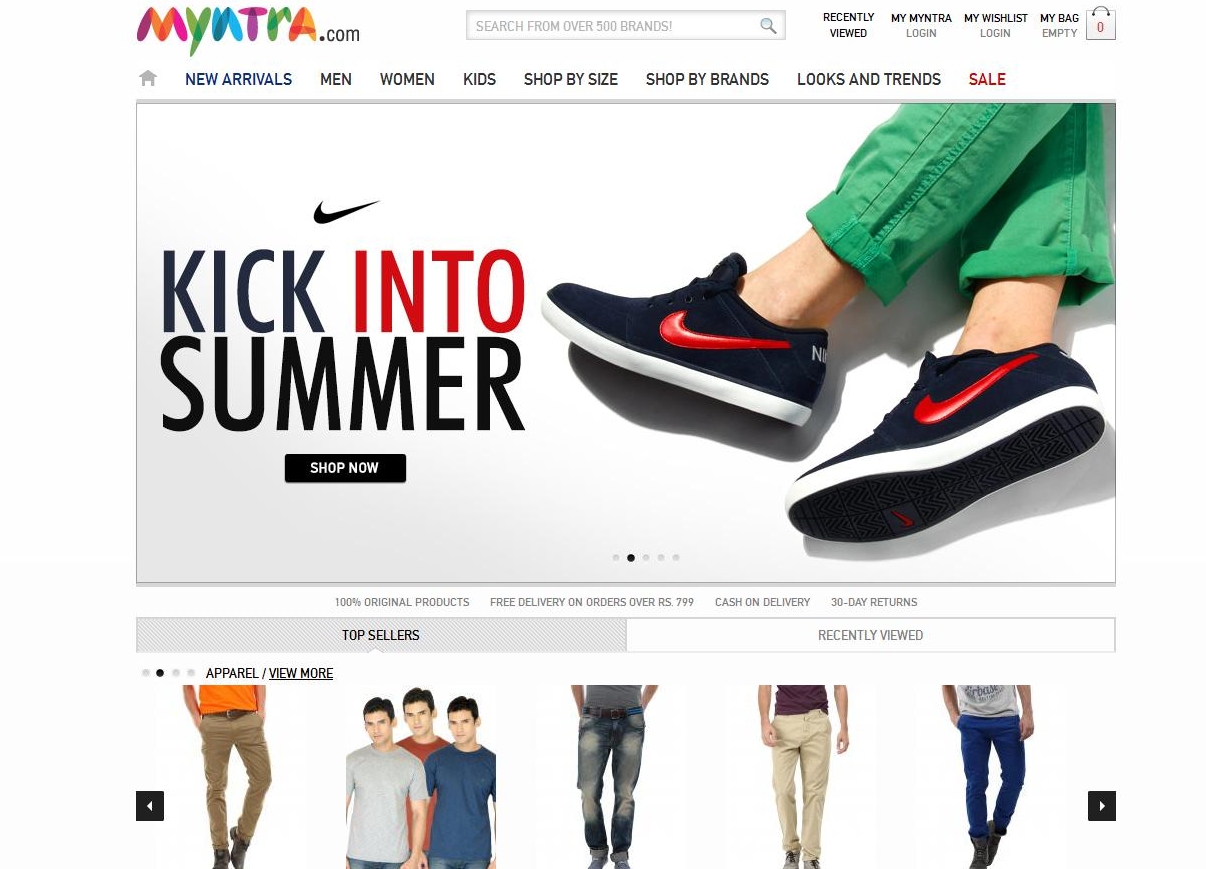The image displays a screenshot from the Myntra website. The Myntra logo is prominently featured in the upper left-hand corner. Centralized at the top of the page is a search bar inviting users to "search from over 500 brands." Nearby in the upper right-hand corner are several interactive buttons labeled 'Recently Viewed,' 'My Myntra Login,' 'My Wishlist Login,' 'My Bag (empty),' accompanied by a shopping bag icon.

Below these elements lies a navigation strip with various categories: 'New Arrivals,' 'Men,' 'Women,' 'Kids,' 'Shop by Size,' 'Shop by Brands,' 'Looks and Trends,' and 'Sale.' 

In the center of the page, there is a promotional section featuring an image of Nike shoes positioned on the right. To the left of the shoes, the text reads "Kick into summer," with a conspicuous 'Shop Now' button beneath.

Further down on the left side, there is a section titled 'Top Sellers' with subcategories like 'Apparel' followed by additional unspecified items. On the right side of this section, there's a 'Recently Viewed' heading. 
Above these sections, a banner states "Free delivery on orders over ₹999."